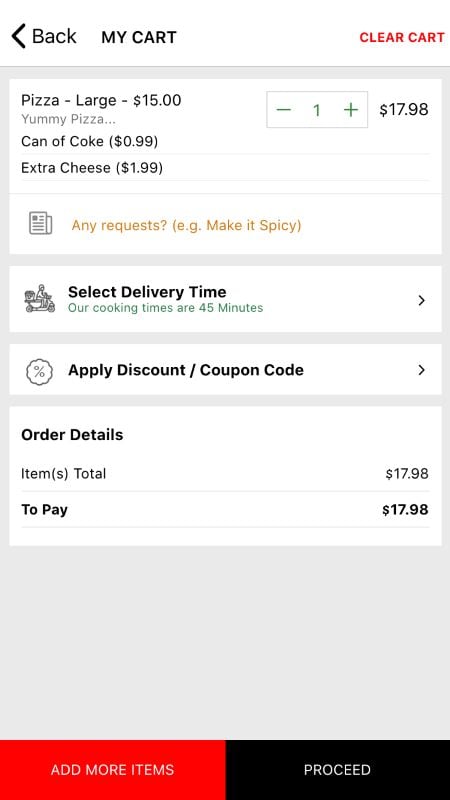The image depicts a mobile-friendly online shopping cart for a food ordering app. The interface mimics the layout of a smartphone screen and displays a summary of the items a user intends to purchase. At the top, there's an item listed as "Pizza Large" priced at $15. The description beneath it, in gray lettering, simply describes the item as "a yummy pizza." 

Following that, in bold black text, there's an item "Can of Coke" priced at $0.99 and "Extra Cheese" for an additional $1.99. Below these items, there is a section labeled "Any Requests?" highlighted in yellow to draw attention. This section includes a placeholder example, "e.g. make it spicy," but the user has left this field blank.

The user has added one pizza to their cart, and with the additional items, the total amounts to $17.98. Further down, a box asks the user to "Select Delivery Time," indicating that typical cooking times are about 45 minutes, with an arrow for expanding options. Another box below this prompts the user to "Apply Discount Coupon Code," where a percentage bubble icon is visible, although this section remains unexpanded.

At the bottom of the screen, there is a summary in a text box stating "Order Details: Items Total $17.98, To Pay: $17.98." Below this are two primary action buttons: a red button for adding more items and a black button for proceeding with the order. The interface's color scheme is predominantly black, gray, and white, with green text for adding item quantities and indicating cooking times, and yellow text for special requests, ensuring these elements stand out.